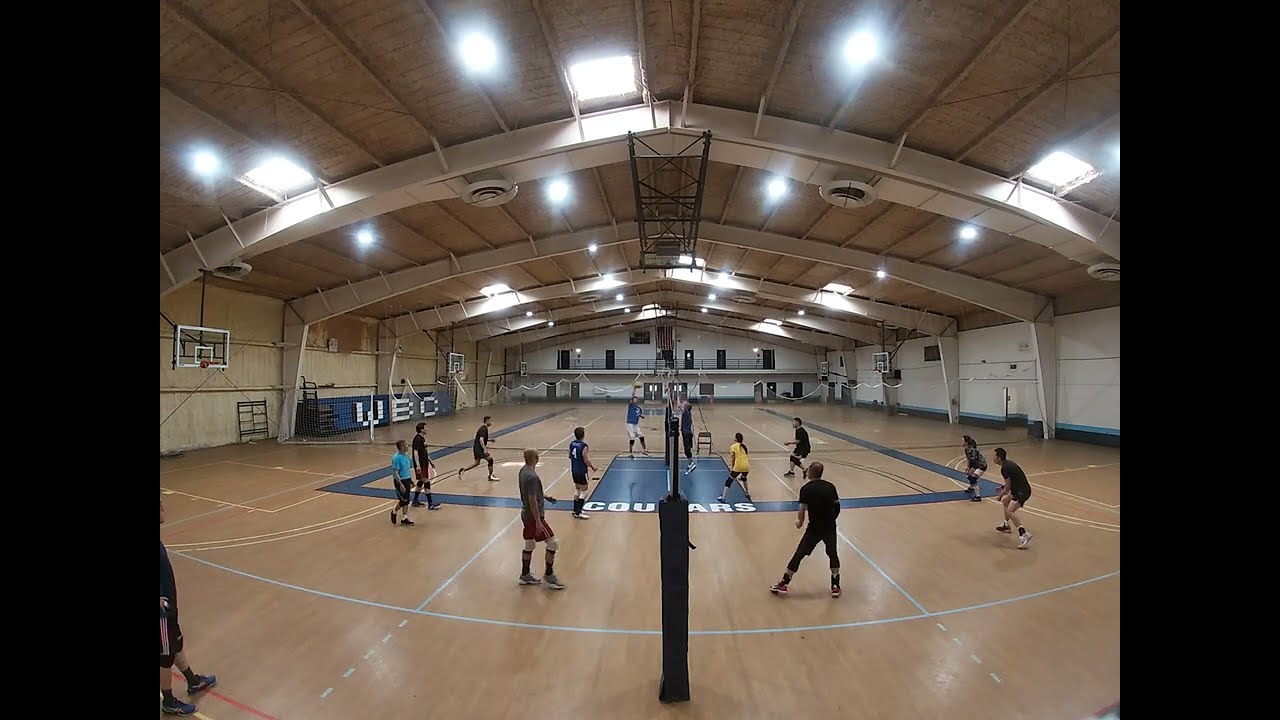The image captures an intense indoor volleyball game with 12 players, six on each side, in a multi-purpose gymnasium. The court's polished wood floor prominently displays the word "Cougars" in white lettering encased in a blue frame. The players, dressed in a mix of dark-colored athletic wear, appear to range in age from teens to men in their 30s. The facility features high ceilings with numerous lights and skylights, brightening the white-walled interior. In the midst of the game, one player is leaping for a spike near the net while an opponent prepares to block him. On the left side, there's an area marked "WBC," spelled out with white blocks on a set of chairs. Additionally, the gym also serves as a basketball court, evidenced by the visible hoops and nets.